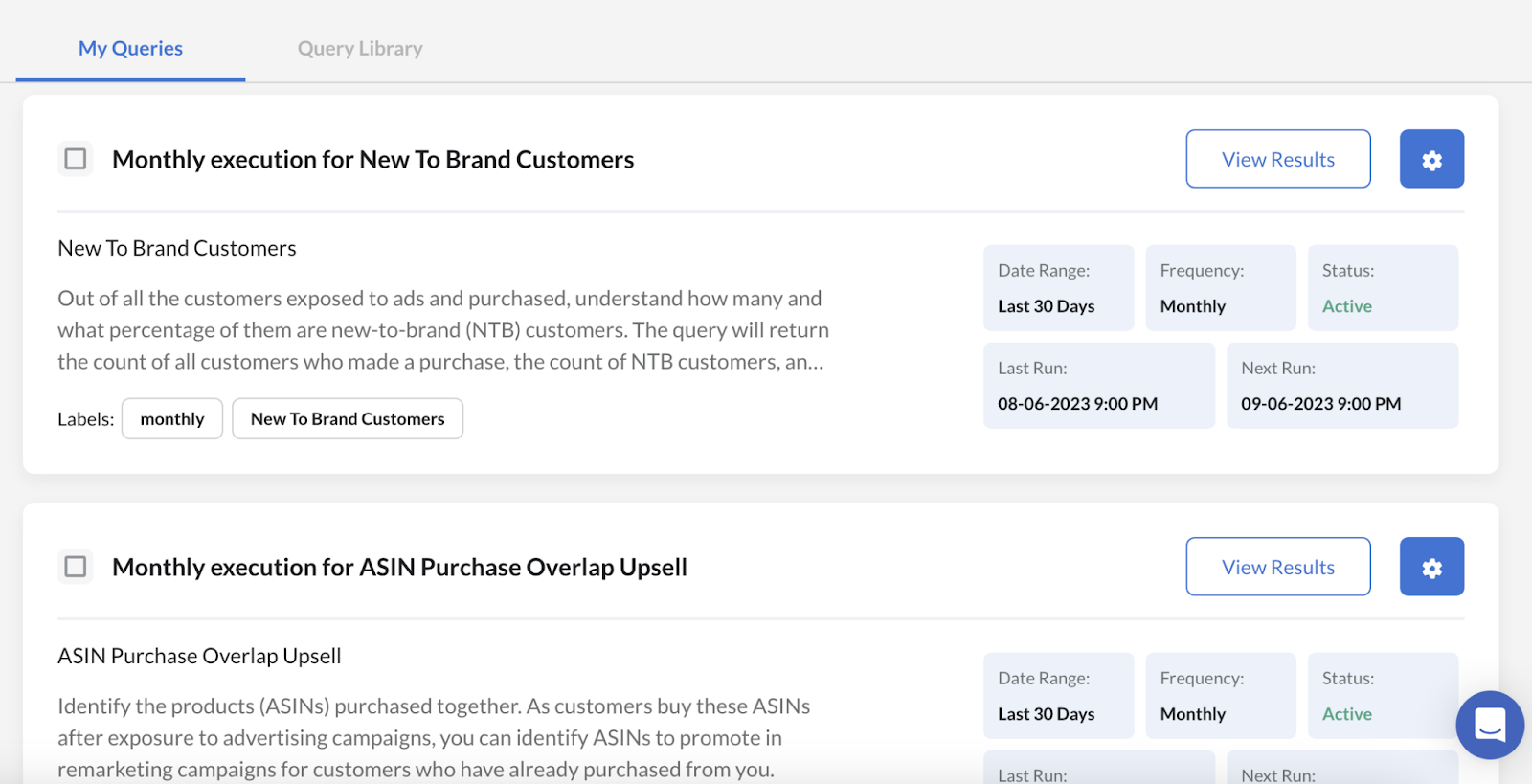This is an image of a screenshot from an unspecified website with a main background color of light grey. The layout features two horizontal, landscape-style white rectangles containing various information. 

In the top left corner of the grey background, the text "My Queries" appears in blue, underlined to indicate the active tab, with "Query Library" written in grey next to it.

**First Information Block:**
The top rectangular white block includes:
- A checkbox in the top-left corner.
- The title "Monthly Execution for New to Brand Customers."
- On the right, a "View Results" button followed by a blue "Settings" button with a white gear icon.
- Below the title, there is additional information about "New to Brand Customers" labeled under "Monthly" and "New to Brand Customers."
  
To the right, there are five light blue rectangles with the following labels:
1. Date Range
2. Frequency
3. Status
4. Last Run
5. Next Run

**Second Information Block:**
The lower rectangular white block includes:
- A checkbox in the top-left corner.
- The title "Monthly Execution for ASIN Purchase Overlap Upsell."
- On the right, a "View Results" button and a blue "Settings" button.
- Below the title, information about "ASIN Purchase Overlap Upsell" is provided.

Similar to the first block, there are five light blue rectangles on the right side with the following labels:
1. Date Range
2. Frequency
3. Status
4. Last Run
5. Next Run

**Additional Feature:**
In the bottom right corner of the image, there appears to be a "Live Chat" option.

The design focuses on clarity and functionality, with essential navigation elements and actionable buttons clearly presented.